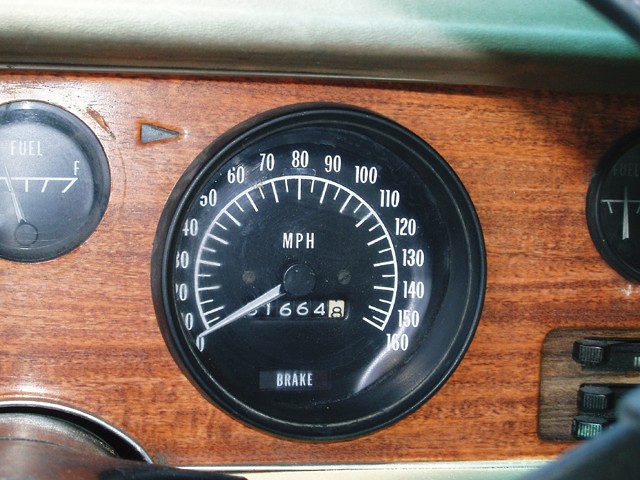This image showcases the dashboard of a vintage car, focusing on two main circular gauges. The first gauge, smaller in size, indicates the fuel level. Adjacent to it is the larger speedometer, which displays speeds ranging from 0 to 160 mph in white ink. The speedometer needle is currently resting at zero. Just above the base of this needle, the letters "mph" are clearly visible, while below it, the odometer reading shows 16648 miles, with the first digit being somewhat ambiguous—either a zero or an eight. Beneath the odometer, the word "brake" is prominently displayed. The background of the dashboard is characterized by a brownish wooden texture, enhancing the vintage aesthetic. Additional dials are spotted in the lower right-hand corner of the image, further reinforcing the classic nature of the car.